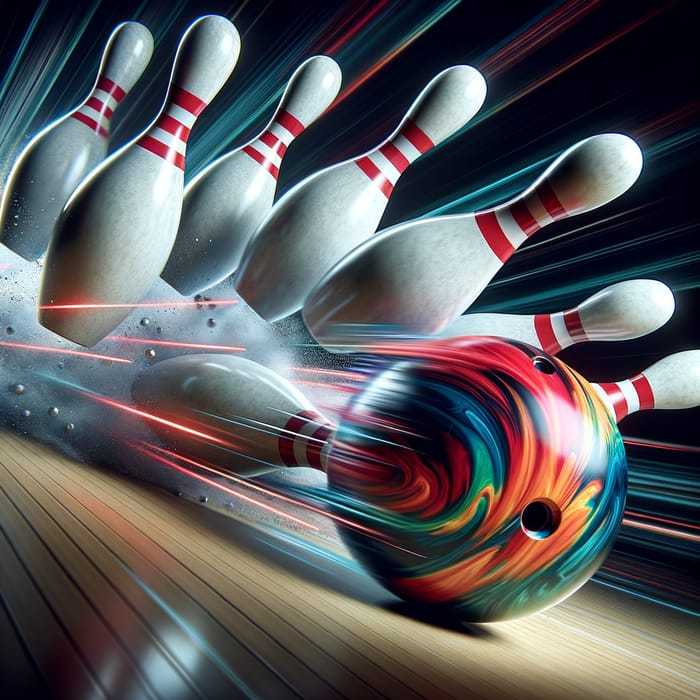The image is a dynamic, computer-generated illustration of a futuristic bowling scene. At the center is a vividly multicolored bowling ball, with swirling hues of red, orange, green, blue, and yellow that give the impression of high speed. The ball has standard finger holes and seems to be in mid-roll, scattering pins everywhere. Surrounding the bowling ball are eight white pins with three red stripes around their necks. Most pins are airborne, with one lying on its side. The background is a striking black, accentuated by light streaks in pink, blue, green, and red that resemble lightning bolts, adding to the sense of motion. The entire scene is set on a wooden lane, with detailed slats contributing to the realism of the illustration.